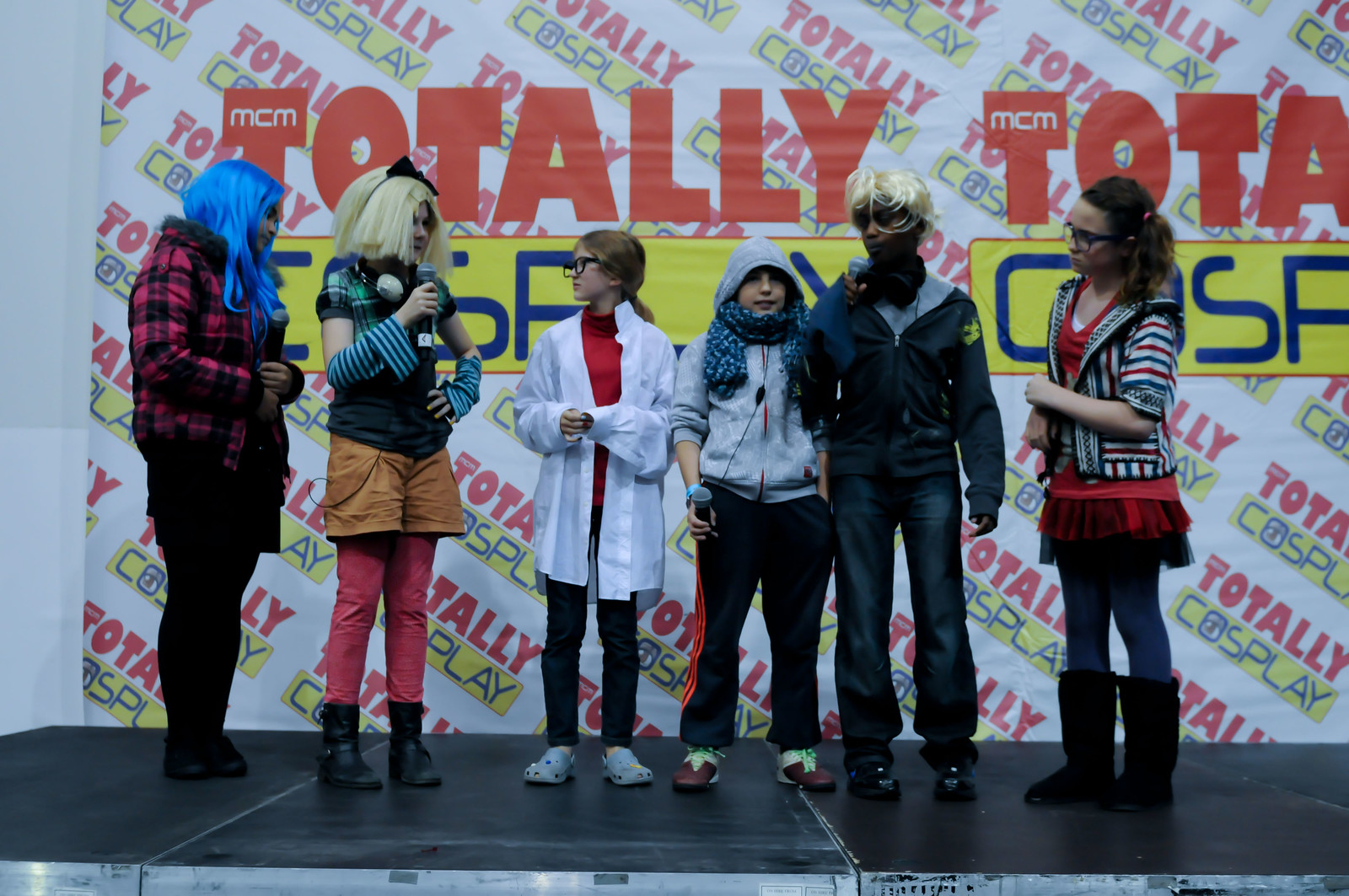The image depicts six children on a stage, each sporting colorful wigs and unique costumes, possibly participating in an event called "Totally Cosplay," as indicated by the repeating signage in the background featuring large, colorful text. Starting from the left, the first child has a long blue wig and wears a red and black jacket. Next to her stands a girl with a shoulder-length blonde wig, holding a microphone, dressed in a black shirt and orange shorts with pink pants. In the middle, there's a girl in glasses wearing a white lab coat, resembling a nurse's outfit. Beside her is another child whose gender is unclear, dressed in a hoodie with a scarf, also holding a microphone. To their right stands a boy with short white hair, wearing jeans and a blue coat. Lastly, on the far right, there's a girl with glasses, tall black boots, and a striped red jacket. All participants appear to be engaged in the event, which seems vibrant and lively, underscored by the playful array of attire and accessories.